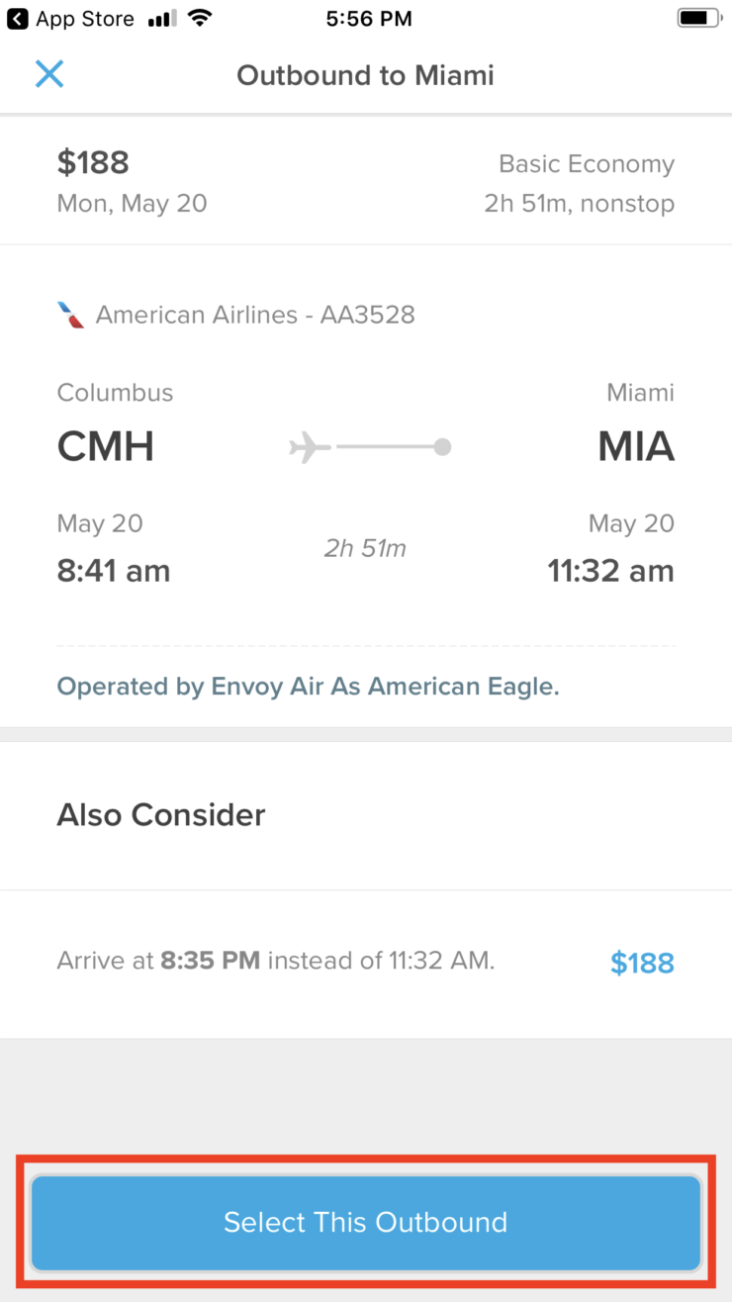**Detailed Caption:**

This image is a screenshot from the App Store, taken at 5:56 PM. The screenshot details a flight itinerary for an outbound trip to Miami. The flight, priced at $188, is scheduled for Monday, May 20th, under a basic economy fare. The journey is a nonstop flight lasting two hours and 51 minutes, operated by American Airlines flight AA3528. The departure is from Columbus (CMH) at 8:41 AM and arrives in Miami (MIA) at 11:32 AM. The flight is operated by Envoy Air under the American Eagle brand. An alternative arrival time mentioned is 8:35 PM instead of 11:32 AM. The screenshot includes a prominent blue rectangular button outlined in red with the text "Select this outbound" for users to proceed with booking this flight.